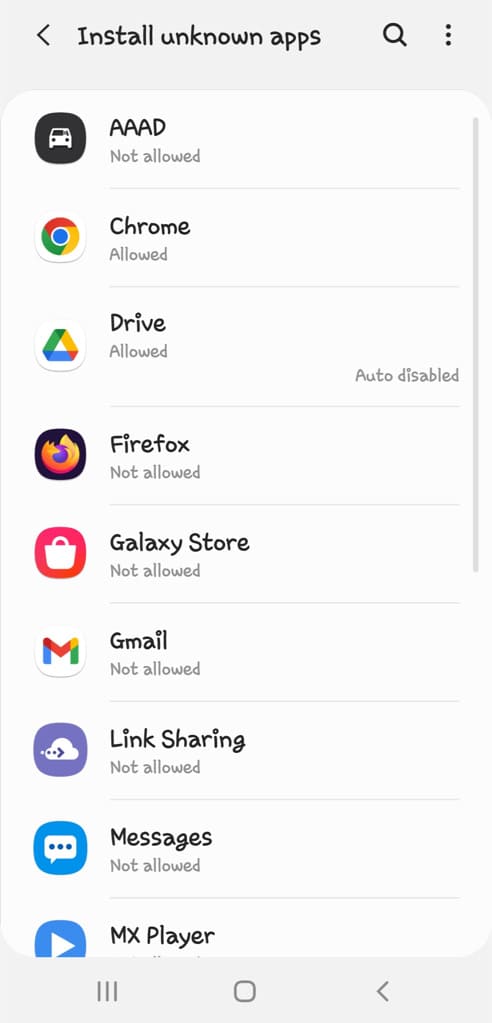The image showcases the settings menu of an Android device, specifically focusing on the "Install unknown apps" section, as indicated by the search input at the top of the screen. The interface exhibits the typical Android layout with navigation icons at the bottom: three horizontal lines, a circle, and an angular back button. The screen displays a list of applications with their respective statuses regarding permission to install unknown apps.

At the top of the list, "AAD" is marked as "Not allowed," followed by "Google Chrome," which is "Allowed." "Google Drive" is also "Allowed" but specified as "Auto disabled." Additionally, "Firefox" is "Not allowed," and the same restriction applies to "Galaxy Store," "Gmail," "Link Sharing," and "Messages." The final visible app is "MX Player."

The layout features a predominantly white and gray color scheme, with each app accompanied by its icon. A vertical scroll bar on the right side indicates the list's scrollable nature. This screen allows the user to manage permissions for installing apps from unknown sources, providing detailed control over each application's settings.